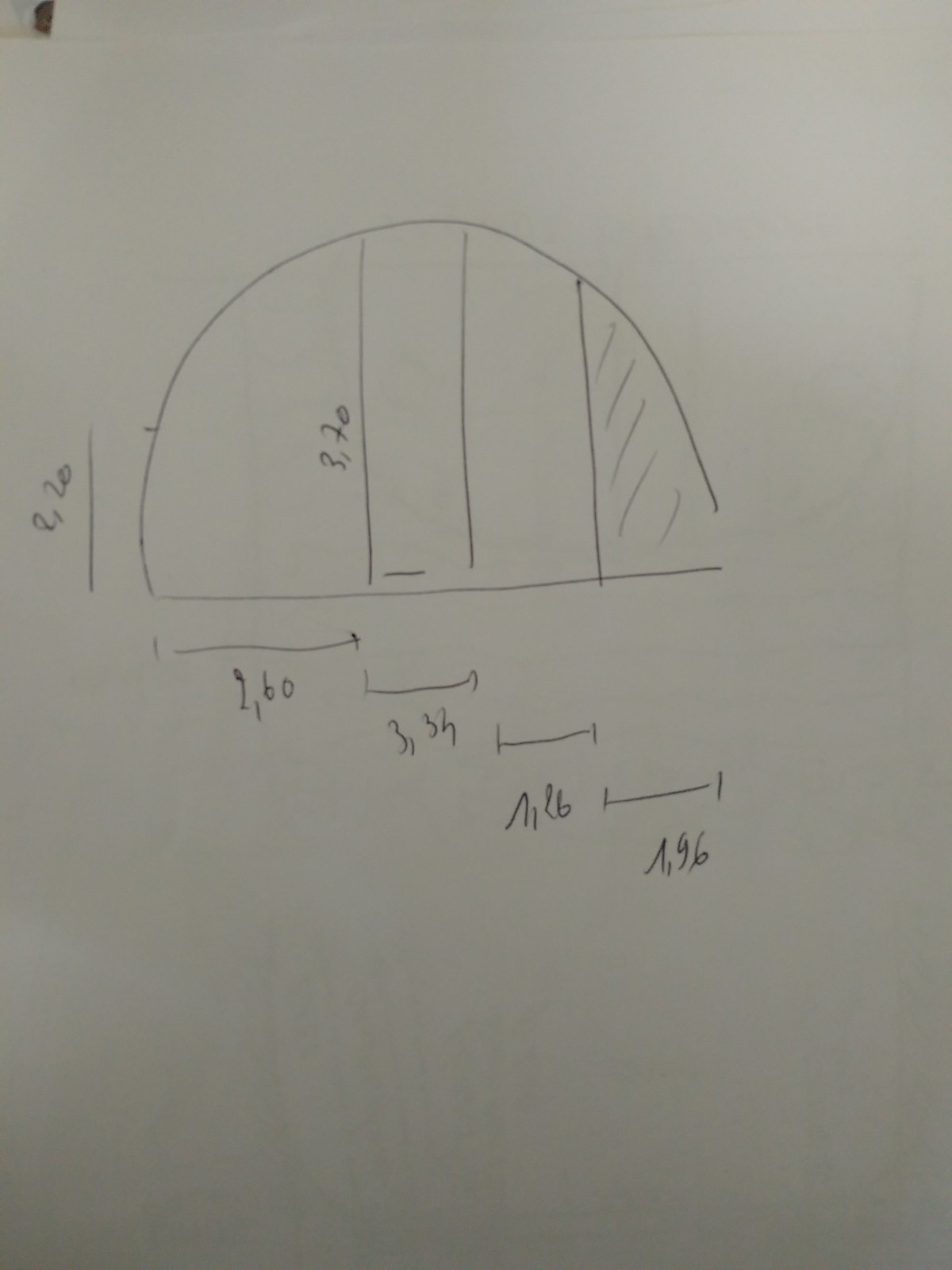This vertically oriented photograph captures what appears to be a white piece of paper or possibly a white wall featuring various sketches and measurements. Central to the image is a horizontal straight line that spans almost the entire width. An arch, resembling a half-moon, connects the two endpoints of this line. Inside the arch, there are multiple lines with notable specifications: one central line marked as three feet, and another vertical line on the right edge of the arch. The space between this vertical line and the curved edge of the arch is detailed with five diagonal dashes.

Beneath this main illustration, to the left, is a shorter vertical line labeled with the number eight. Further down, additional horizontal lines are drawn with arrows extending from them, each ending with tabs. These lines stack downward in a stair-like fashion and have numbers written beneath each step, adding another layer of complexity to the sketch.